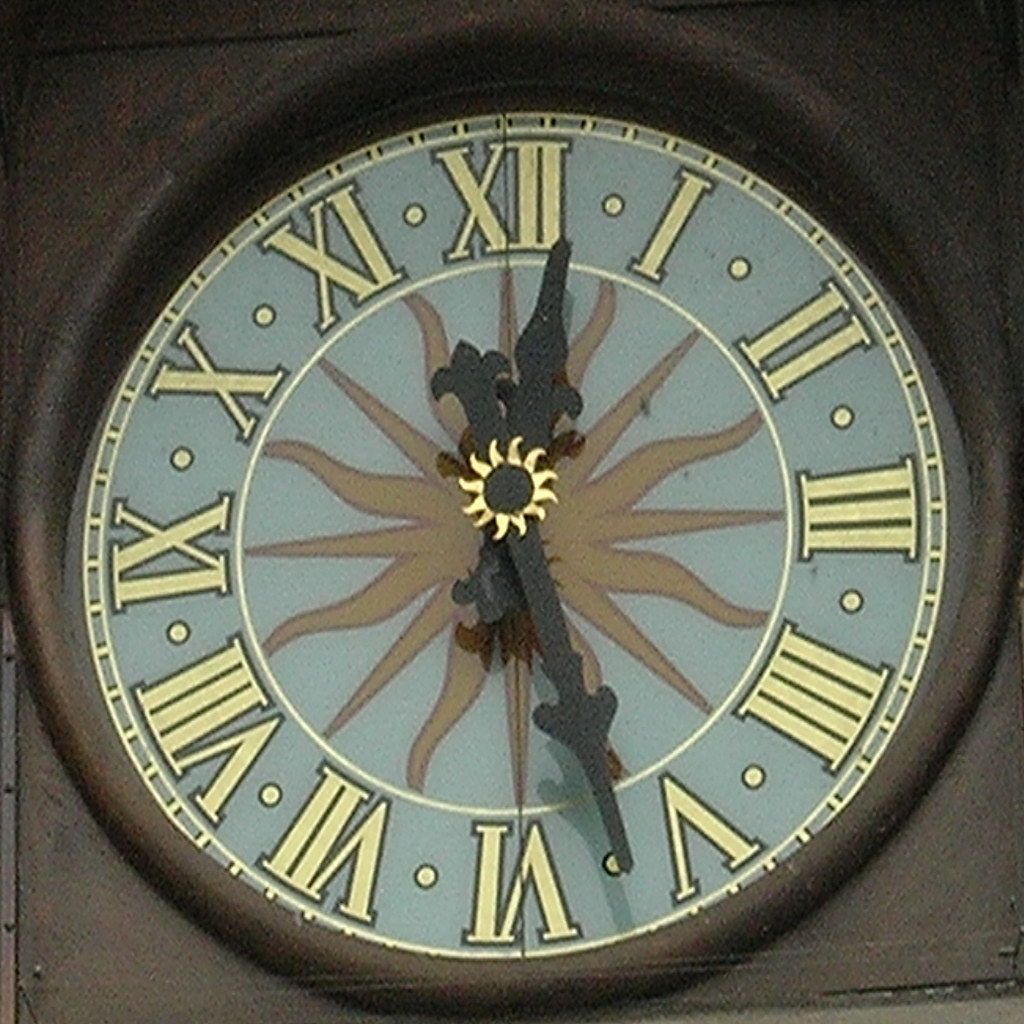This image showcases a circular clock hanging on an outdoor wall, surrounded by what appears to be gray concrete. The clock's frame seamlessly blends with its background due to its similar gray hue. The clock face is a serene baby blue, adorned with Roman numerals in a soft beige color. Adding a unique touch, the center of the clock features an intricate brown design resembling the delicate arms of an octopus, radiating outward. The clock's hands are ornate and black, pointing to the time 12:28.